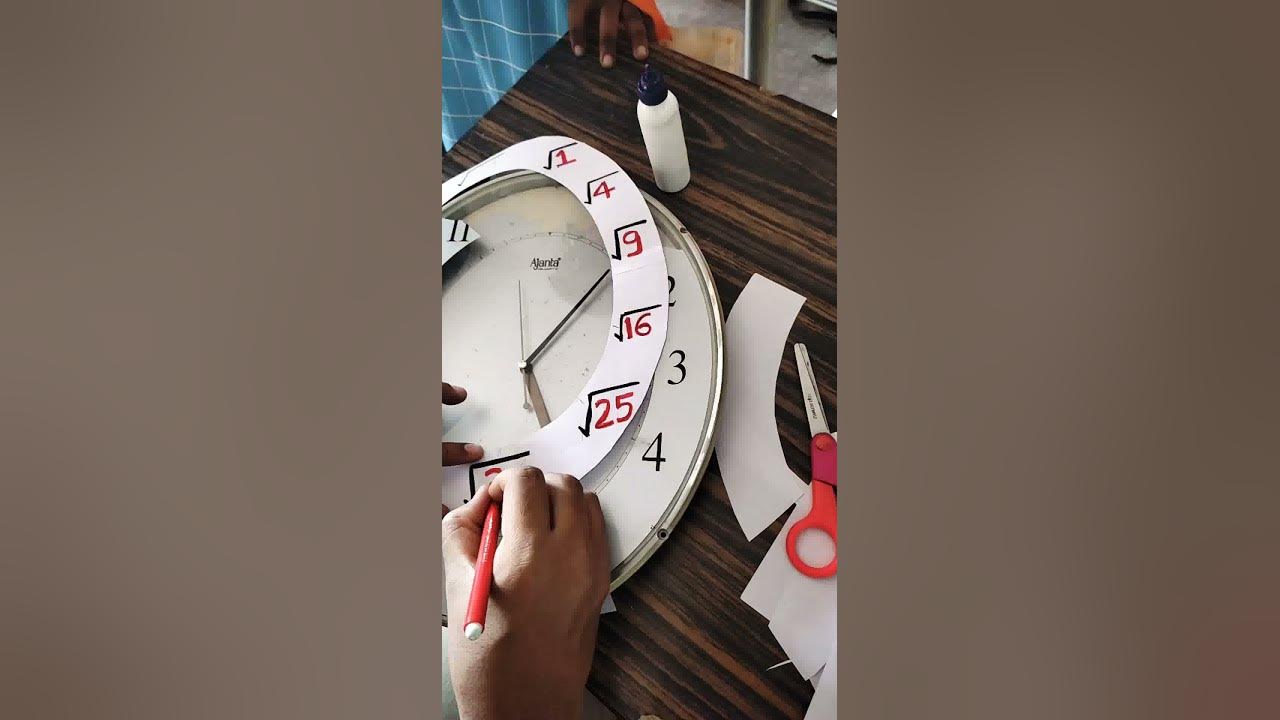In this meticulous photograph, a craft project is in progress on a wooden desk. A clock is being used as a stencil to outline and draw intricate details. The setting includes a blue fabric with a thin plaid pattern, suggesting that a woman might be involved in this delicate task. Her presence is indicated by three fingers visible at the top left corner of the desk. The main hands at the bottom, dark-skinned and deft, maneuver a piece of paper cut to match the dimensions of the clock. The individual is precisely drawing square roots on the paper, aligning them with the corresponding numbers on the clock face. This detailed work involves calculating and illustrating square roots that equate to each number typically found on a clock, merging mathematical elegance with artistic precision.